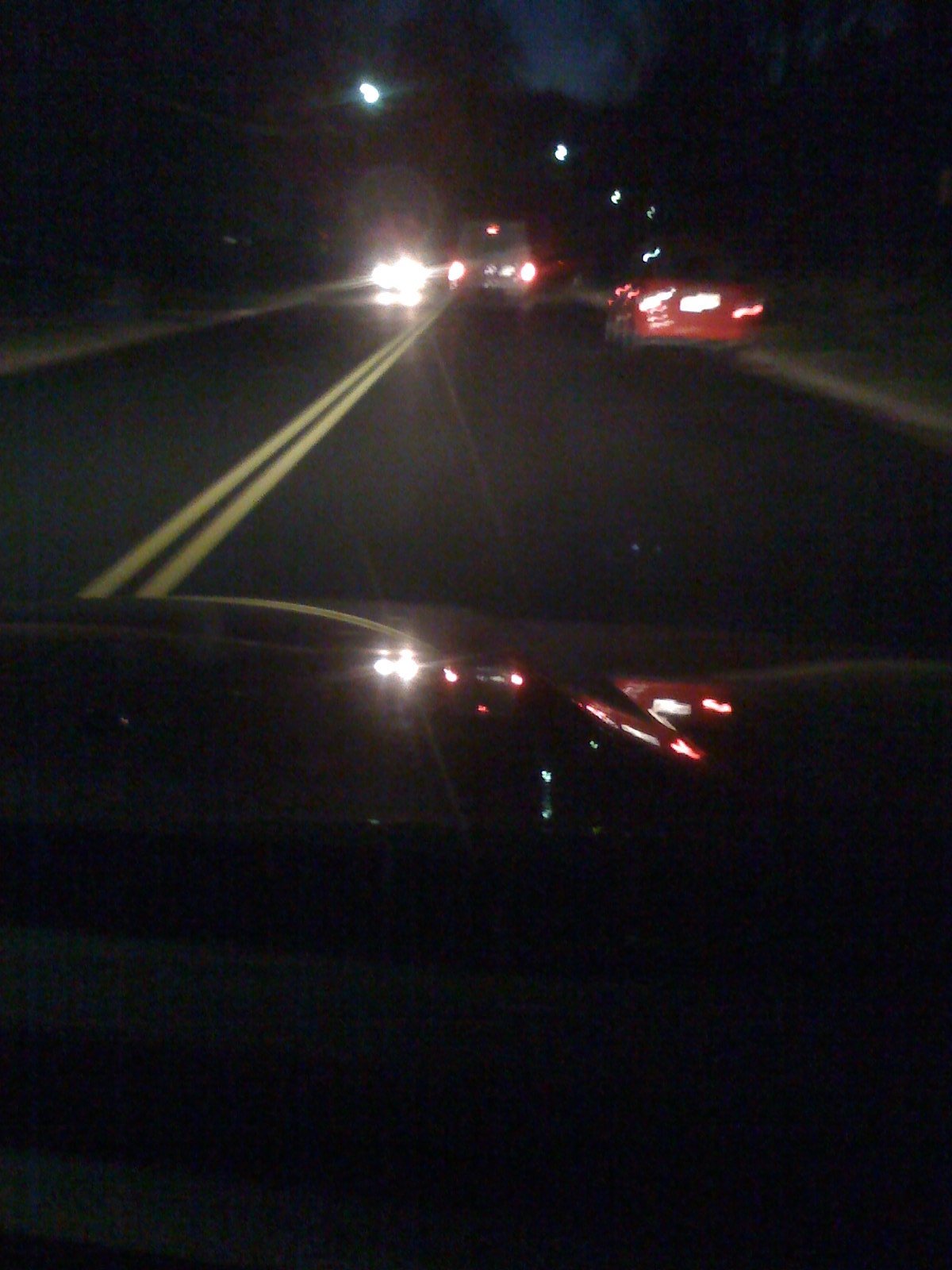From the perspective of someone either driving or riding in a car, this photograph captures a scene as viewed through a car's windshield. The image might have been taken using a dashboard camera and then extracted as a still image. A two-lane road stretches ahead and we see both oncoming traffic and vehicles moving in the same direction as the car from which this photo is taken. The closest vehicle in the same lane appears to be a red car, while the other vehicles' details remain indiscernible due to blurriness. It’s night time, and the scene is dimly illuminated by a few sparse streetlights and the headlights of the oncoming cars. Shadowy trees line the sides of the road, further emphasizing the darkness of the night. The image does not contain any text.